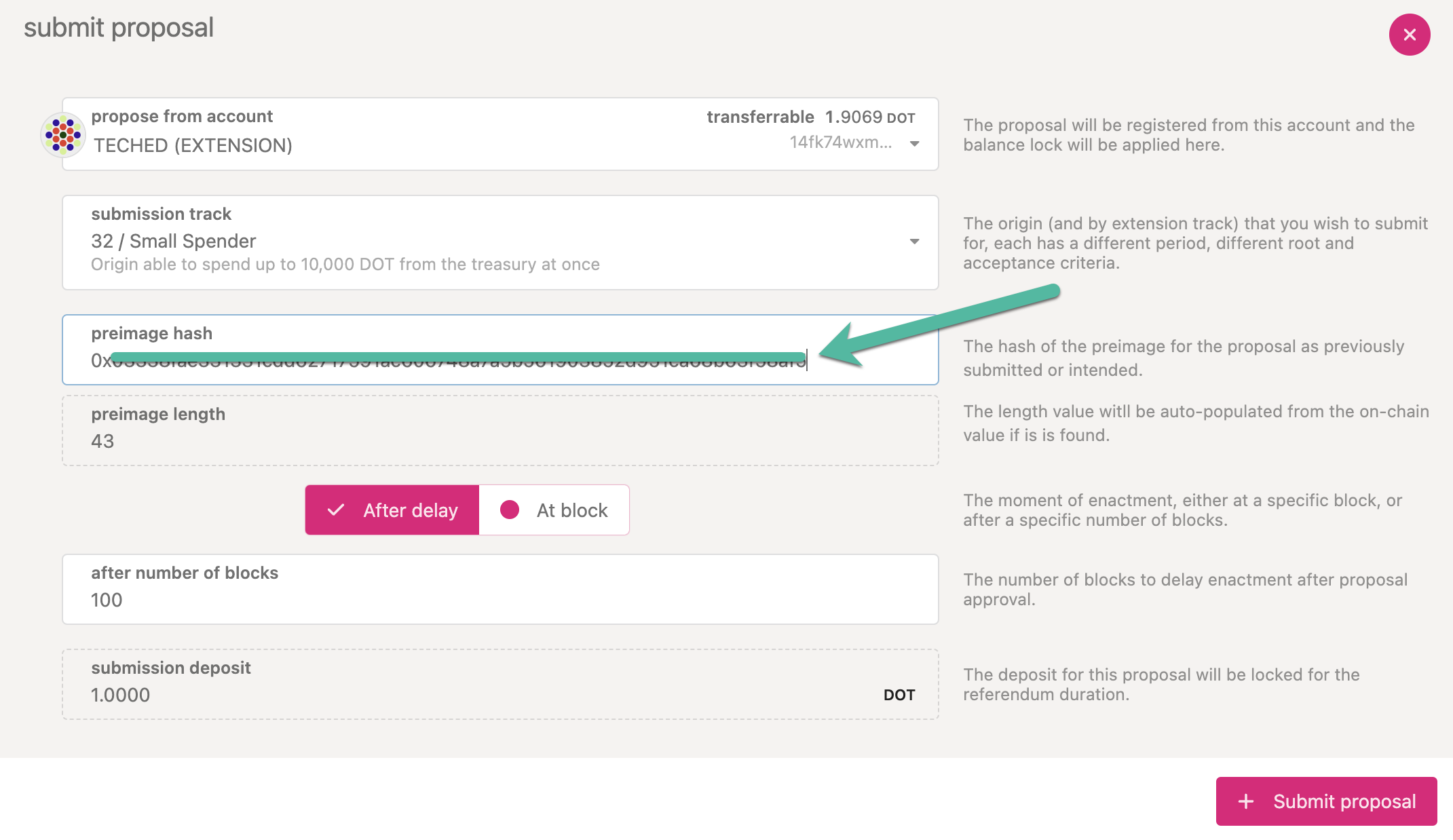This image captures a detailed screenshot from a 'Submit Proposal' page on someone's computer screen. The background is predominantly a light grayish-tan color. At the top, the screen displays the text "Propose from account," followed by "TECH-ED extension." Below that, there is a field labeled "Submission Track," containing the text "32/Moss Bender."

In the middle section, a teal line overlays a lengthy alphanumeric string in the "Pre-image hash" field, indicating a code or hash value. Adjacent to this hash is an arrow in the same teal color, pointing leftward towards the line.

Further down the screen, there are sections highlighted in pink. One such area is labeled "After delay," featuring a white check mark within the field. Next to it is another section tagged "At block," marked by a pink circle.

Finally, at the bottom of the screenshot, there is a pink button labeled "Submit Proposal," which includes a plus sign.